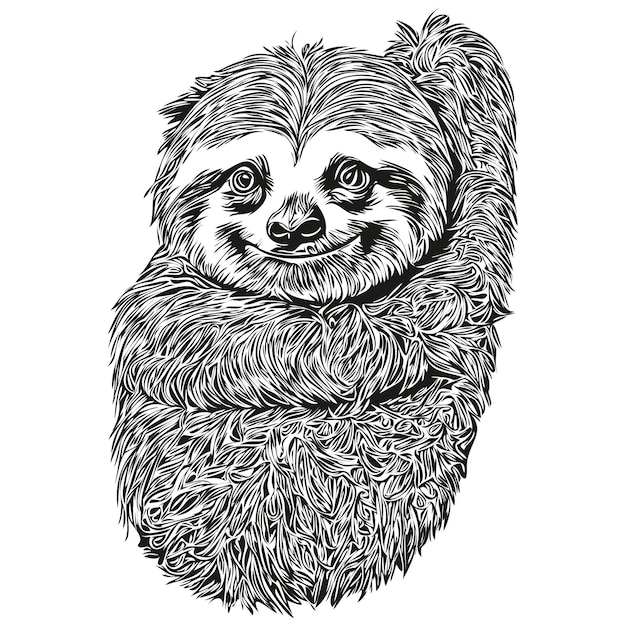This black-and-white pen and ink illustration features a charming and whimsical depiction of an animal that most closely resembles a sloth, but with fantastical elements drawing a parallel to a baby Wookiee. The creature is curled up in a snug little ball, embracing itself with its arms wrapped around the left side of its head. Its fur, meticulously detailed with an almost wave-like texture, appears parted down the center of its head. The endearing figure looks directly at the viewer with large, round, kind eyes, a somewhat crooked nose, and an adorable little grin. The overall effect of the detailed and evocative illustration captures a delightful blend of realism and fantasy, inviting viewers into a playful and heartwarming interpretation of a baby Wookiee or a cuddly sloth.